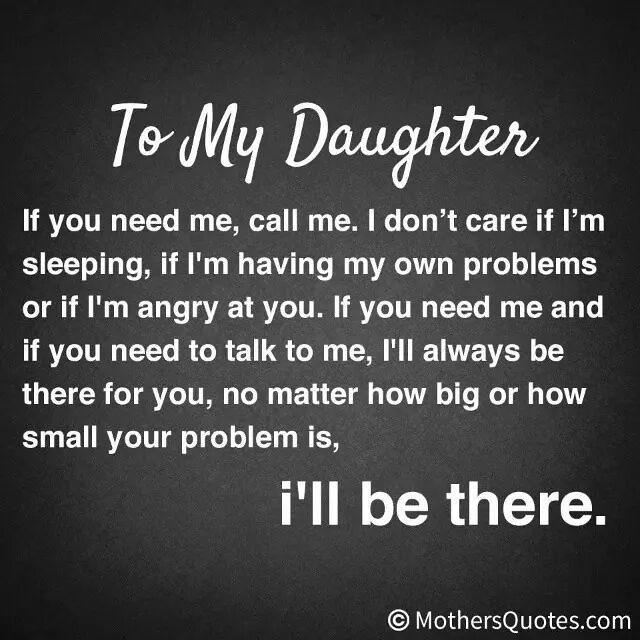The image is a heartfelt message set against a gradient background that transitions from a dark grey at the edges to a lighter grey towards the center. The text is primarily in white, with "to my daughter" written across the top in cursive. The rest of the message reads, "If you need me, call me. I don't care if I'm sleeping, if I'm having my own problems, or if I'm angry at you. If you need me, and if you need to talk to me, I will always be there for you, no matter how big or how small your problem is. I'll be there." In the lower right-hand corner, the image is copyrighted by mothersquotes.com. This touching note emphasizes a parent's unwavering support for their daughter.